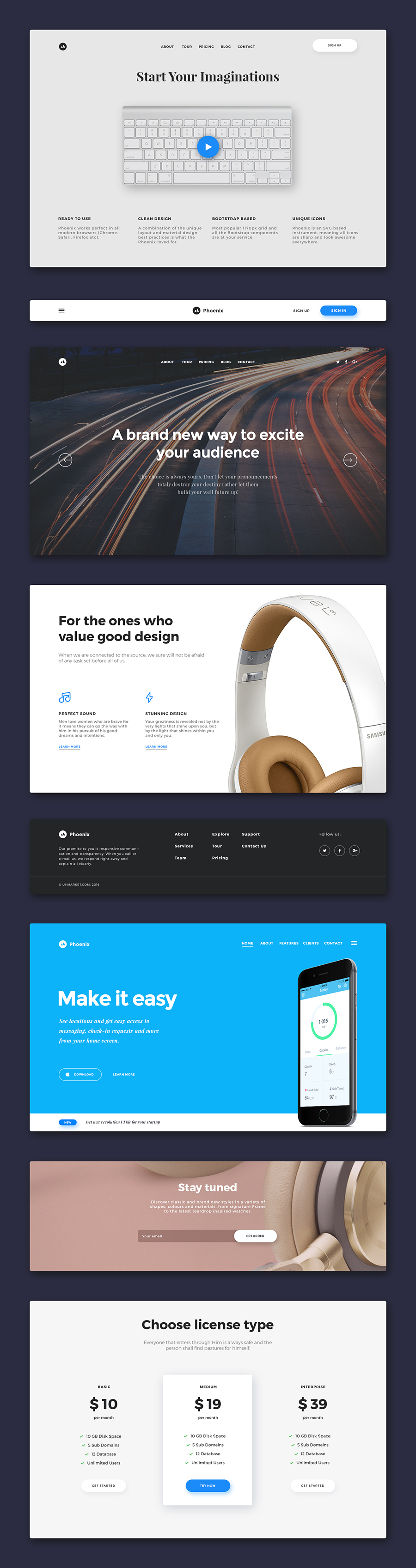This image is a screenshot likely taken from a website or as a pop-up advertisement. The tall, blue rectangular screen is divided into six distinct sections, each representing a different advertisement, although the text is quite small and difficult to read. 

1. The first section features an image of a computer keyboard with the tagline "Start Your Imagination."
2. The second section displays a photo of traffic on a highway and reads "A Brand New Way to Create Your Audience."
3. Subsequent sections include advertisements for headphones and a mobile device, among other products that are not easily identifiable due to the tiny text.

Each section seems to promote a distinct product or service, combining diverse visuals and headlines aimed at attracting different types of consumers.